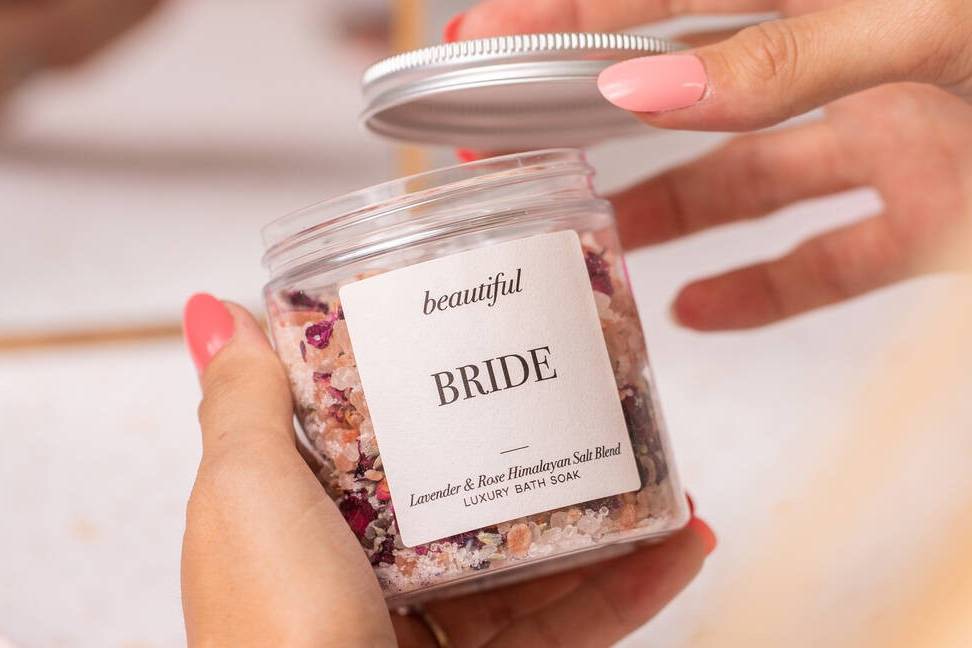The image is a horizontal rectangle featuring a close-up of a woman's hands holding a small jar. The woman's left hand, adorned with a wedding band and long, pink fingernails, grasps the jar in her palm. Her right hand is in the process of lifting the silver lid off the jar. The jar itself contains a colorful blend of granules, including various shapes and sizes of white, pink, and purple salts, suggesting it's a bath salt blend. The white label on the jar has black text that reads, from top to bottom: "BEAUTIFUL," followed by a space, then "BRIDE" in larger font, and below that, "LAVENDER AND ROSE HIMALAYAN SALT BLEND, LUXURY BATH SOAK." The background of the image is white and blurred, focusing attention on the product. The product appears to be a luxury bath soak designed for a bride to use before her wedding.